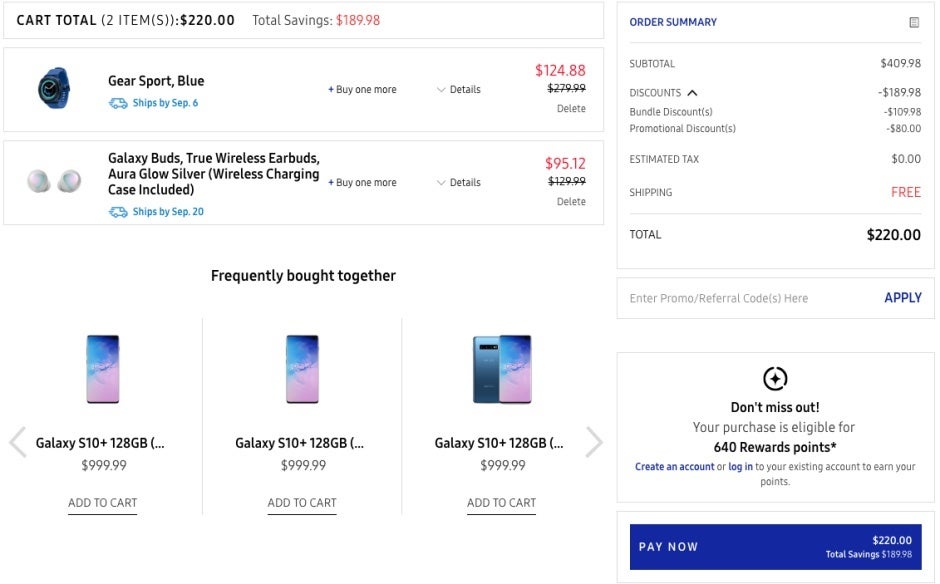The screenshot captures the checkout page of a desktop website displaying the details of a purchase. On the left side of the screen, the cart summary shows two items with a combined total of $220. Highlighted in red text, the total savings amount to $189.98. The two items in the cart are:

1. **Gearsport Blue**, priced at $124.88
2. **Galaxy Buds, True Wireless Earbuds, Aura Glow Silver with Wireless Charging Case**, costing $95.12

Below the cart summary, there is a suggestion for frequently bought together items, featuring three Galaxy S10 Plus devices, each priced at $999.99.

To the right, the order summary details the costs and discounts applied. The subtotal for the items was initially $409.98. Discounts totaling $189.98 were applied, broken down into a bundle discount of $109.98 and a promotional discount of $80. The estimated tax is zero, and shipping is free. The final total for the purchase amounts to $220.